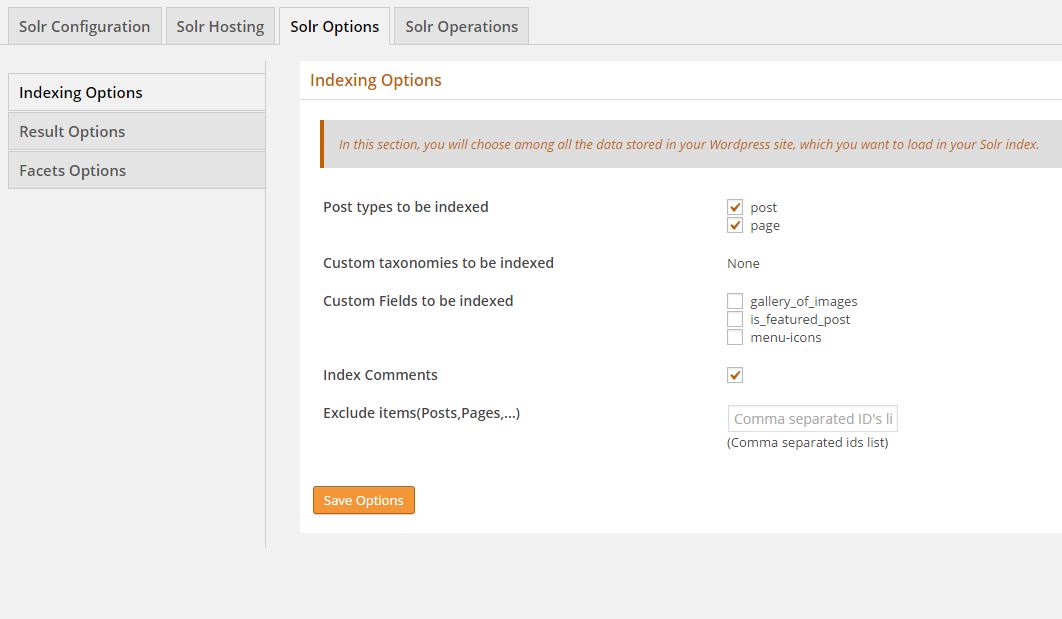The website interface displays configurations for SOLR, indicated in gray text at the top left corner. Just below, it features navigation tabs labeled "SOLR Hosting," "Options," and "Operations." The left sidebar lists categories including "Indexing Options," "Result Options," and "Facets Options."

Within the main content area, the "Indexing Options" section is highlighted in orange. Below this header, an explanatory gray bar has orange text stating, "In this section, you will choose among all the data stored in your WordPress site which you want to load into your SOLR index."

Following this, black text outlines specific settings:
- **Post Types to be Indexed**: Post and Page
- **Custom Taxonomies to be Indexed**: None
- **Custom Fields to be Indexed**: Gallery of Images, Featured Post, and Menu Icons.

Additionally, the option to "Index Comments" is available, accompanied by a red-checked box. Users can exclude items by entering post page IDs in a comma-separated list under "Exclude Items". Finally, a prominent orange bar labeled "Save Your Options" is positioned toward the bottom of the webpage for users to save their configurations.